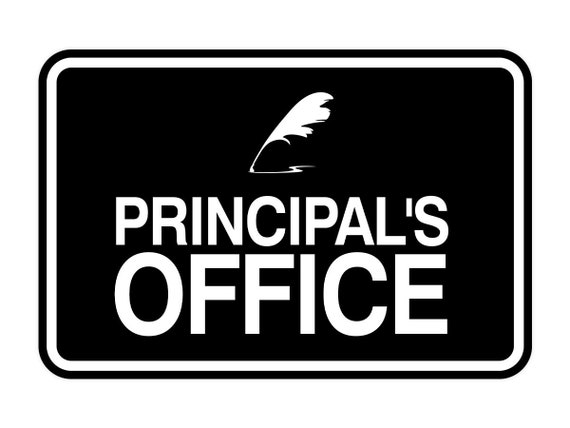The image depicts a black and white sign, bordered first by a thin black line, then a thin white line of equal width. The primary background of the sign is black. At the top center, there is an illustrated feather, resembling an ink quill, with a curved line trailing behind it, suggesting old-style writing. Below this, in bold, white letters, it reads "PRINCIPAL'S OFFICE," with "OFFICE" appearing larger than "PRINCIPAL'S." The entire sign gives a nostalgic feel, evoking memories of school days. The sign is fairly simple and likely intended to be mounted on the door of a principal's office, and measures approximately six inches wide by three inches tall. No additional elements or colors are present in the image.